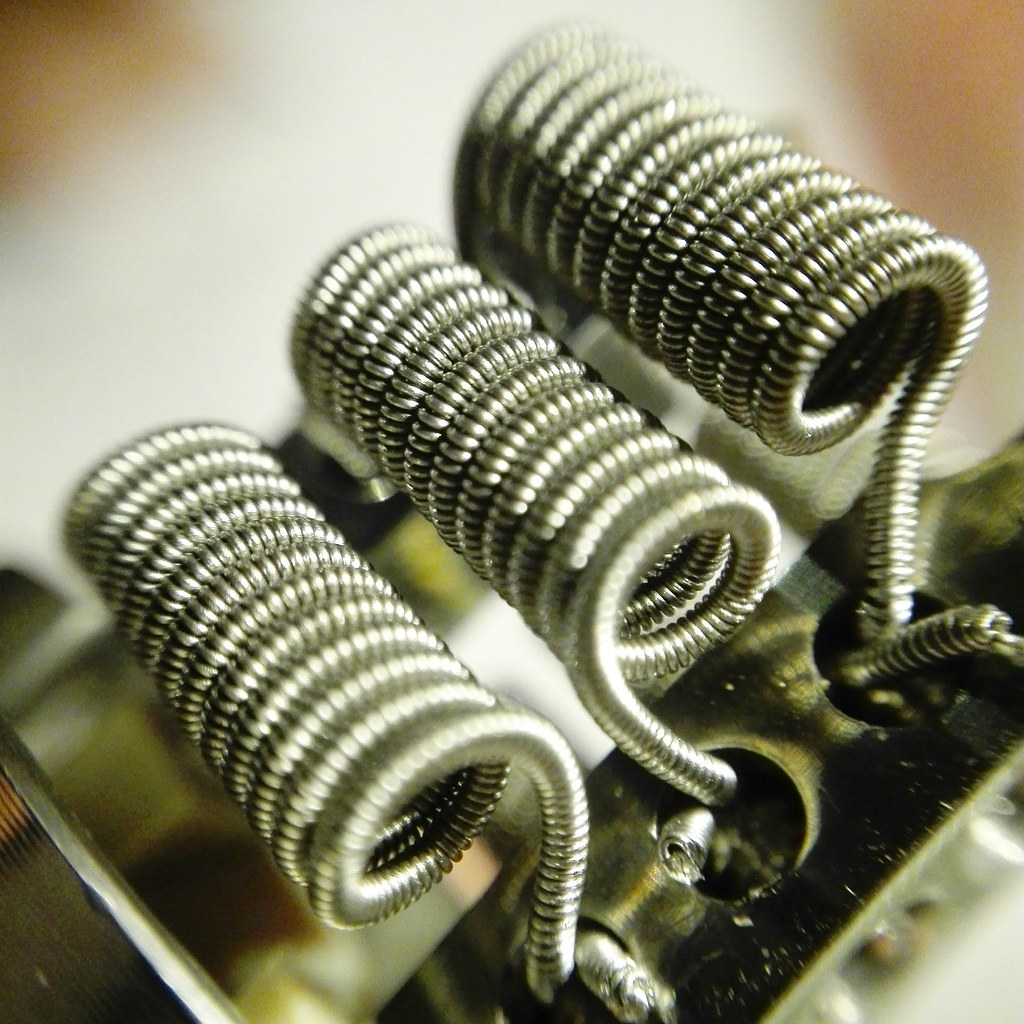The image is an indoor, extreme close-up color photograph showcasing three stainless steel coils that are part of a heating mechanism, possibly from a hair dryer or toaster oven. The coils are made from tightly wound spiral wire, with each coil containing between 10 to 15 loops. The coils are arranged diagonally, with the ends pointing right and left, leading to a metal plate with three holes at one end. Another metal plate is visible at the opposite end. The front portion of the coils is in sharp focus, reflecting light, while the background appears as a light blur. A diagonal metal strip is also visible, starting from the lower portion of the image and extending out of the frame to the right. The overall setup suggests that the coils are designed to heat up when an electric current passes through the plates, emitting heat as part of an electronic device.